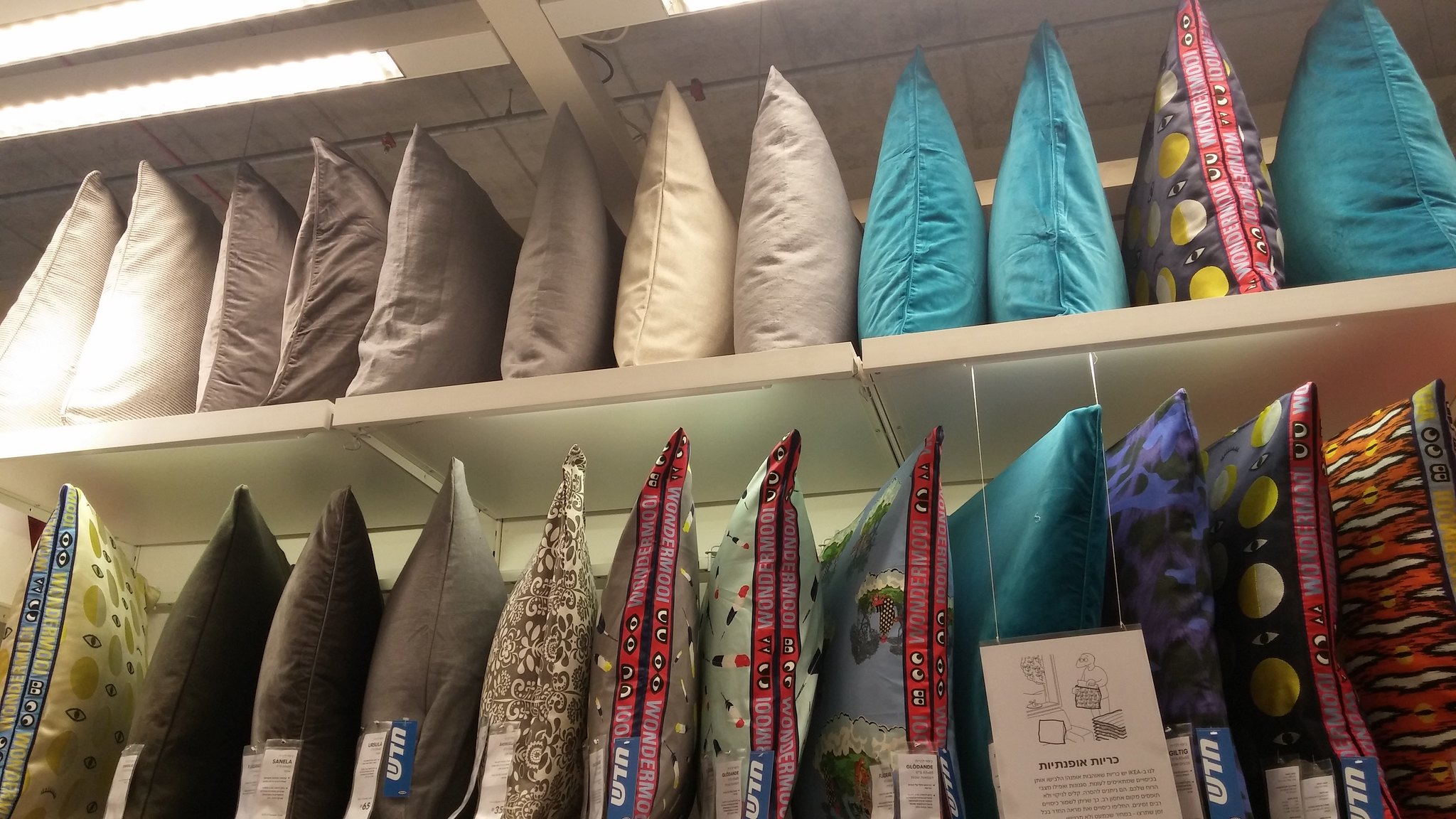The photograph captures two shelves of decorative throw pillows inside a store, viewed from an angle that suggests the shelves are above eye level. The store's ceiling, with long bright lights, creates a well-lit scene that highlights the diverse collection of pillows. The top shelf displays an array of pillows: starting from the left, there are two white pillows, four brownish-gray pillows, followed by a cream-colored pillow, a tan pillow, two teal pillows, and a unique pillow featuring a pattern of the phases of the moon and eyeballs. This shelf concludes with another teal pillow. Below, on the bottom shelf, there's a contrasting pillow with a white background adorned with green circles and eyeballs, instead of the gray background and yellow circles. This shelf also holds two black pillows, a gray pillow, a gray and white paisley-patterned pillow, and three others with assorted fabric patterns possibly depicting blow pops and globes. There's also a teal pillow, a dark blue pillow with a floral pattern, another moon phases and eyeballs pillow, and a pillow with a U.S. Southwestern style pattern. A poster with writing, possibly in Hebrew, hangs in front of the shelves, alongside price tags attached to the pillows, indicating their cost.